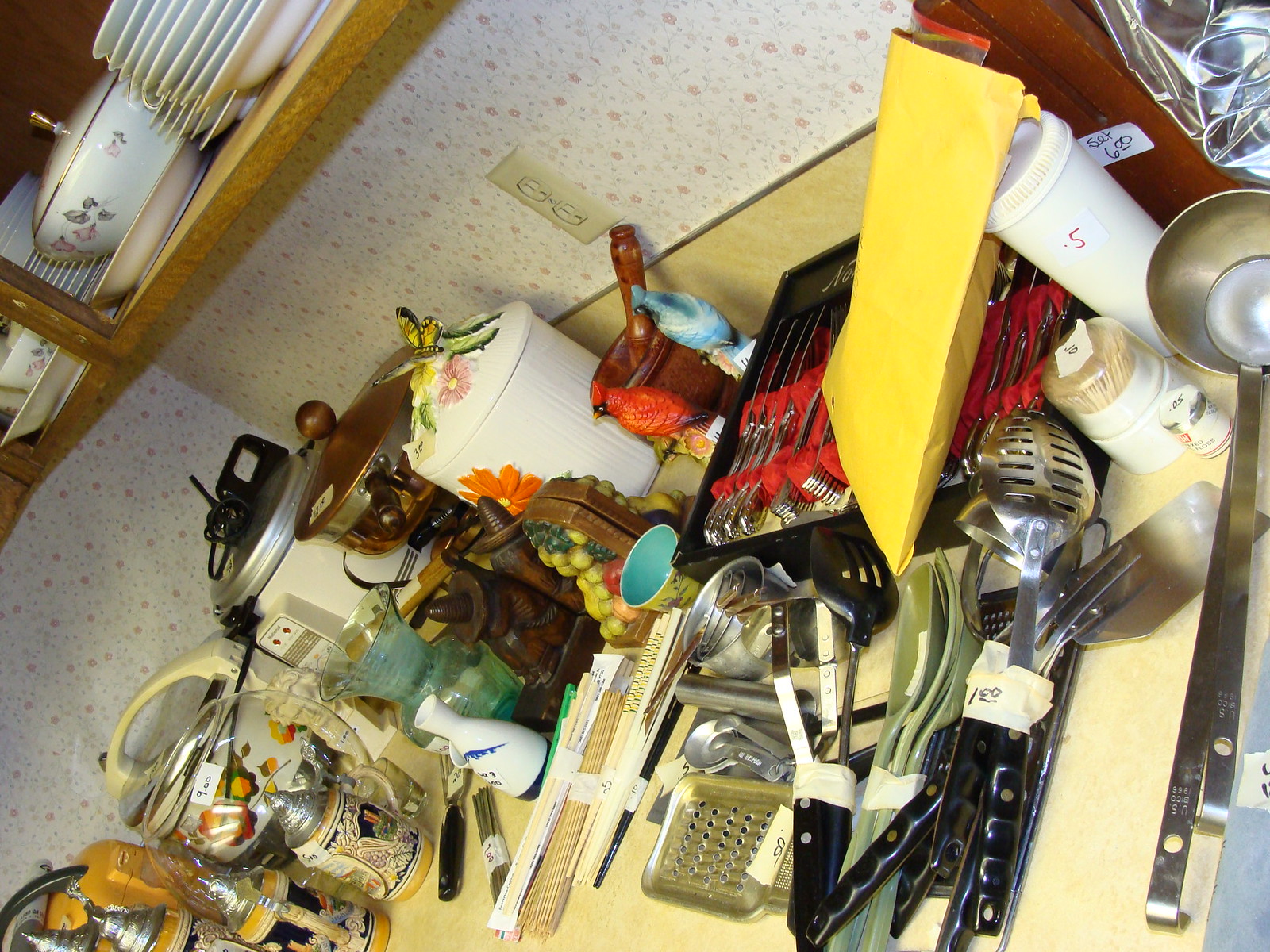A slightly tilted photograph captures a charming kitchen scene. The centerpiece is a beige wooden table, adorned with a multitude of kitchen utensils and implements. Arranged haphazardly, the table hosts a container filled with various spoons and cutlery, standing separate from an array of spatulas and ladles. Pots and containers with lids are clustered together, creating a mélange of metallic and plastic kitchenware. Notably, a mortar and pestle rest among the assortment. 

In the background, a white wall patterned with small pink flowers adds a touch of quaintness to the setting. A white electrical outlet is visible on the wall, directly below a glass-front cabinet. Inside the cabinet, neatly arranged china plates and a pot with a lid are on display, contributing to the kitchen's homely atmosphere.